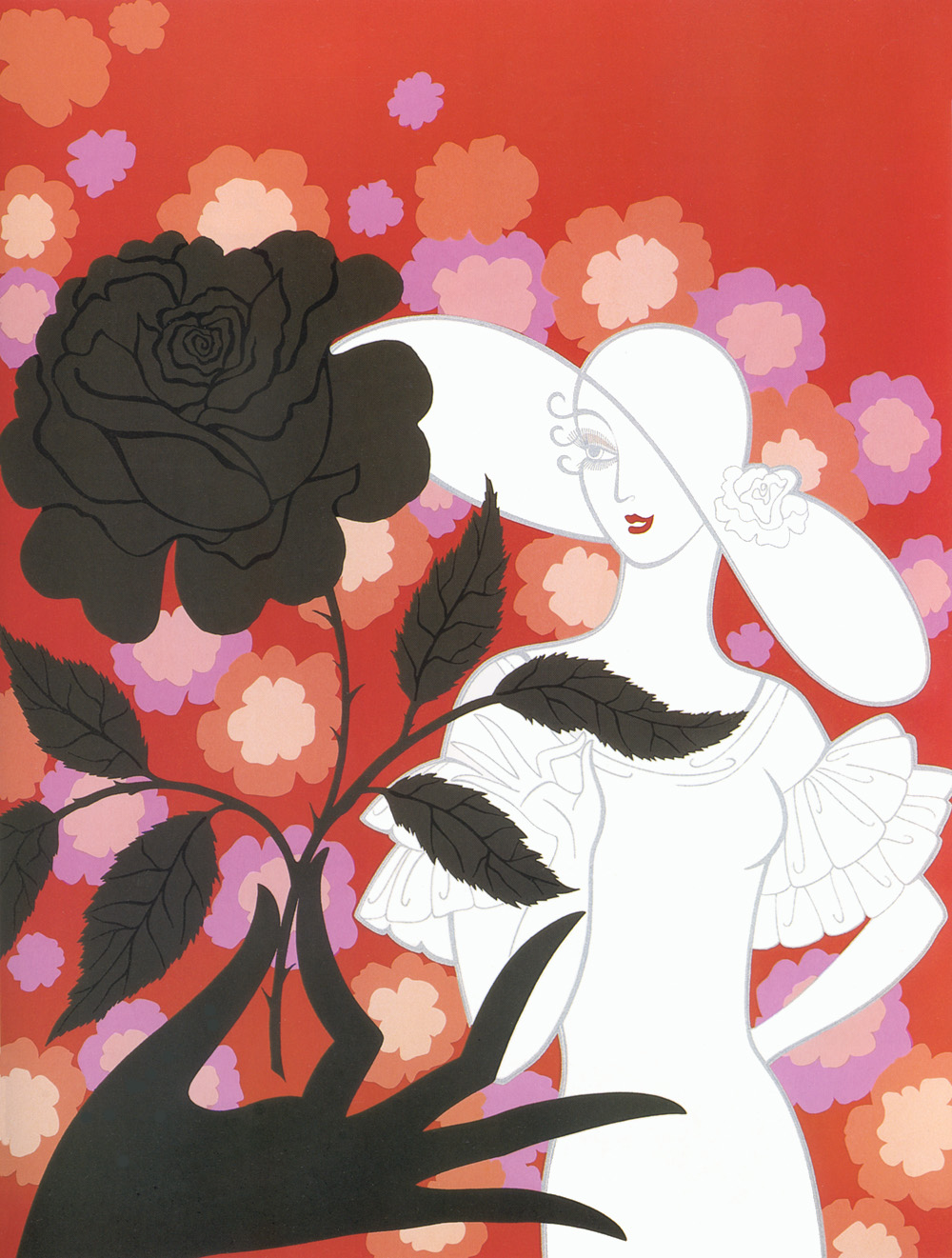The painting, titled *Black Rose* by the artist Erte, is a stunning Art Nouveau illustration with a vibrant and colorful backdrop. The portrait-oriented illustration showcases an elegantly dressed woman, entirely in white, standing on the right side of the image. Her attire includes a large floppy hat adorned with a flower, a layered, ruffled white dress, and red lips which strikingly contrast her monochrome appearance. The woman's delicate features are punctuated by her visible eye and defined by gray outlines, with tendrils of grayish hair peeking out from under her hat. She appears to be in her 30s and gazes to her right.

In the foreground, a shadowy, dark rose is held delicately by a feminine hand, depicted in blacks and grays, clasped between the forefinger and thumb, with the other fingers elegantly spread. This rose is being presented to the woman, and it serves as a focal point of the piece, drawing attention to the interplay of light and shadow. The background is a bright orange, filled with a multitude of flower illustrations in hues of orange, lavender, and peach, with yellow and hints of brown at their centers. These floral elements cascade diagonally from the top left corner to the bottom right, enhancing the overall dynamic and colorful composition of the artwork. The contrasting elements of the white woman and the dark rose, set against this vibrant backdrop, create a visually arresting and richly detailed scene.